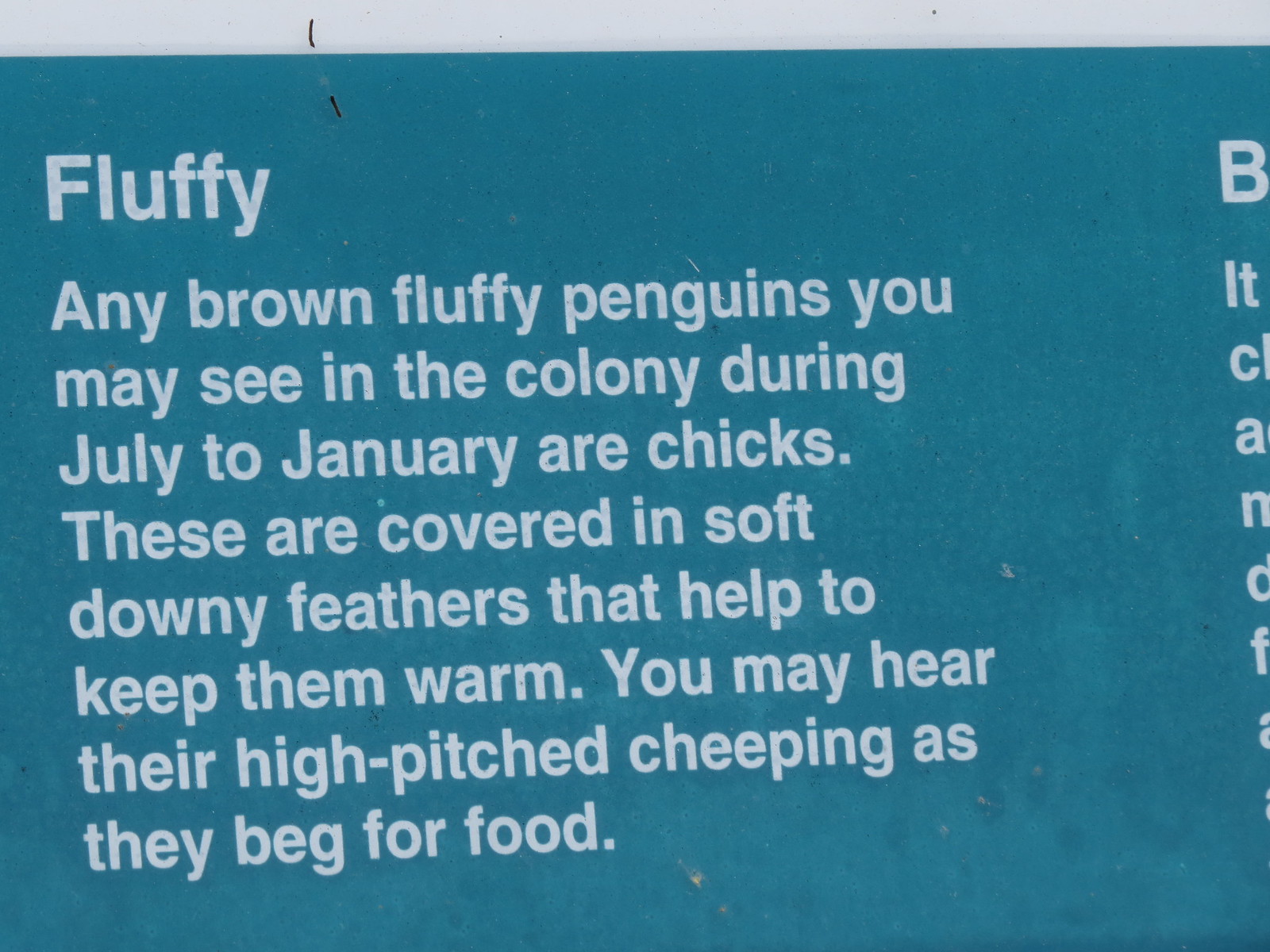The image features a blue rectangular piece of paper with white lettering. The majority of the text is centrally aligned, with a clear and prominent title at the top that reads "Fluffy." Below the title, a detailed paragraph states, "Any brown fluffy penguins you may see in the colony during July to January are chicks. These are covered in soft downy feathers that help to keep them warm. You may hear their high-pitched cheeping as they beg for food." The text is confined to the central and left portion of the image, with the right edge showing a partial letter hinting at truncated text beyond the visible paragraph. The robust blue background covers the entire image, except for a lighter blue border at the top. Overall, the image is simple and monochromatic, featuring no other elements or imagery.